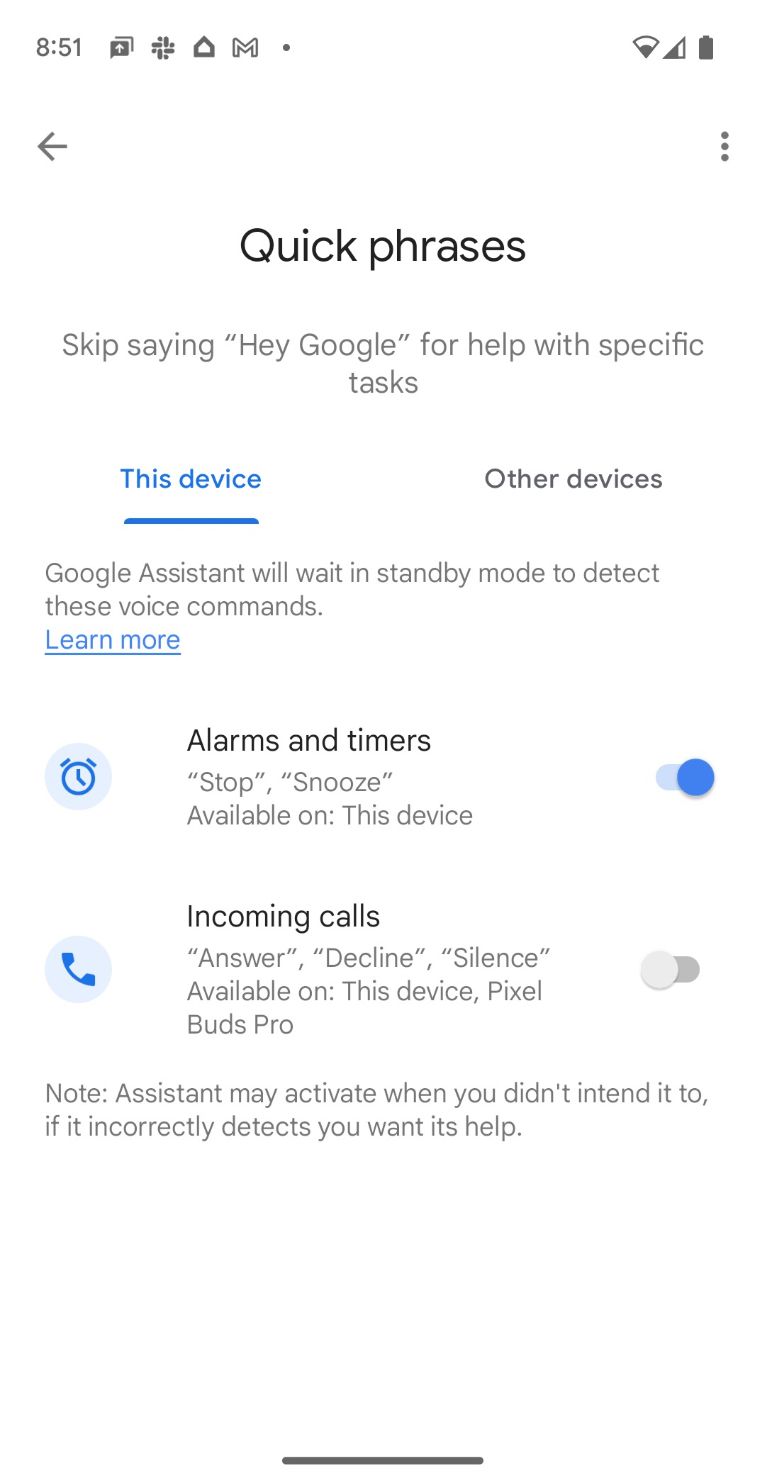The image appears to be a screenshot of a cell phone's settings page, specifically focused on the "Quick Phrases" feature within the Google Assistant settings.

In the upper-left corner, the time is displayed as 8:51 alongside standard icons indicating Wi-Fi, cellular data, and battery status on the right-hand side. There are also three vertical dots in the upper-right corner, likely representing additional menu options.

Centered at the top of the screen in bold black text is the title "Quick Phrases." Below this title, a description in light gray reads, "Skip saying 'Hey Google' for help with specific tasks." The phrase "Hey Google" is enclosed in quotation marks.

On a navigation bar, "This Device" is highlighted in blue and underlined, indicating the current selection, while "Other Devices" appears in gray, showing it is not currently selected. An explanatory note in gray text below the navigation bar states, "Google Assistant will wait in standby mode to detect these voice commands." The phrase "Learn more" is underlined and written in blue, suggesting a hyperlink to additional information.

The settings options are listed as follows:

1. **Alarms and Timers** (accompanied by a small clock icon):
   - Description: "Stop" and "snooze" commands available on this device.
   - Status: Enabled, indicated by a blue toggle switch positioned to the right.

2. **Incoming Calls** (preceded by a small blue phone icon within a light blue circle):
   - Description: "Answer", "decline", and "silence" commands are available on this device and Pixel Buds Pro.
   - Status: Disabled, represented by a grey toggle switch positioned to the left.

A final note in gray text at the bottom of the settings list states: "Assistant may activate when you didn't intend it to. If it incorrectly detects you want its help, normally if it sounds like that." This serves as a caution about potential accidental activations.

No further text is present in the image.